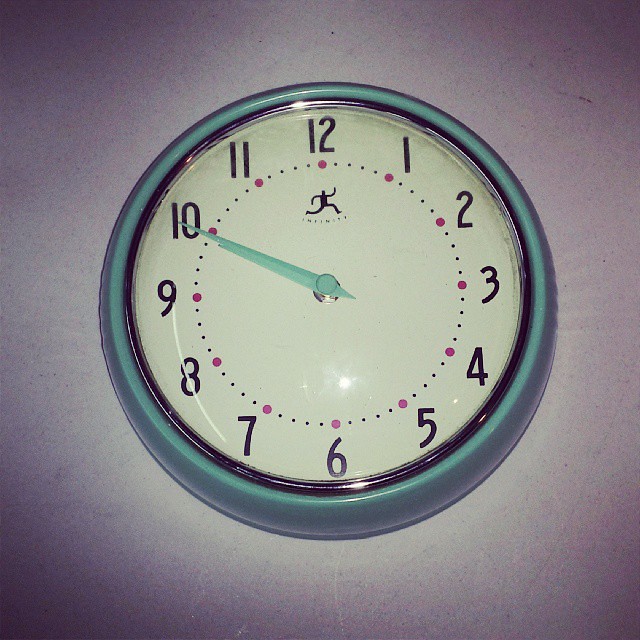This photograph features a circular analog wall clock with a striking teal frame. The clock face is a clean, crisp white, adorned with bold black numbers for easy readability. Matching the frame, the hour and minute hands are also teal, creating a cohesive and stylish look. Adding a unique touch, the clock displays a small logo of a running man along with the word "Infinity" and tiny tick marks beneath it, subtly emphasizing the concept of endless time.